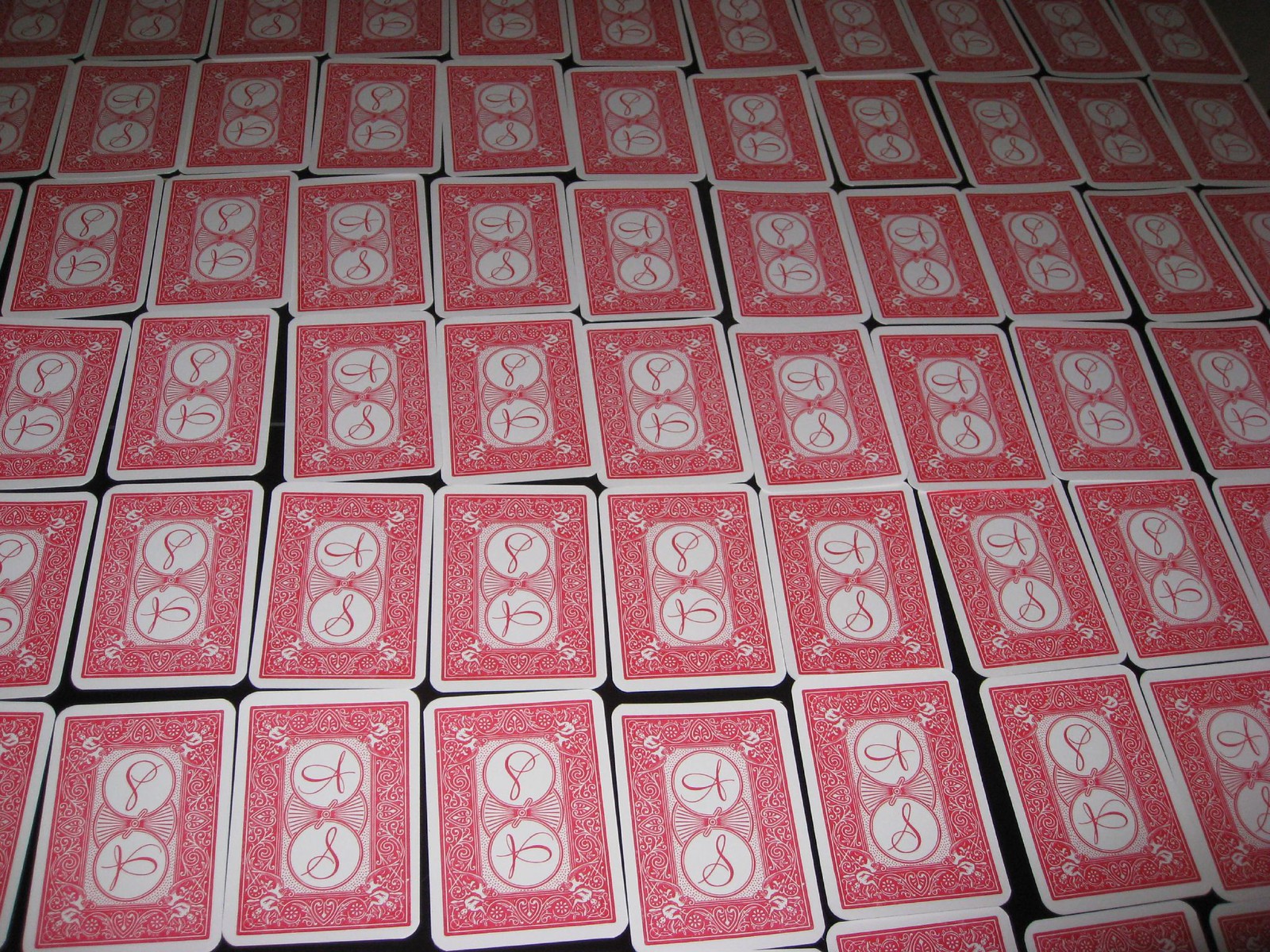An image set against a black background displays an expansive array of playing cards meticulously spread out in horizontal rows, each row stretching from the left to the right edge of the frame. There are at least eight rows, consisting of five cards each, with additional rows partially visible along the edges of the photograph. The backs of the cards are red, framed with an intricate white design. Each card's center features a light pink rectangle containing two white circles adorned with a delicate red filigree that resembles the letters "A" and "S" in cursive.

While the cards are predominantly aligned in straight rows, variations are apparent: some spaces between cards are slightly wider and a few cards are subtly tilted either to the left or right. The uniform black background peeks through these gaps, emphasizing the arrangement. Notably, all cards are facing downward, displaying only their decorated backs. It appears that the entire deck of cards has been laid out on the surface, creating a visually striking and meticulously organized display.